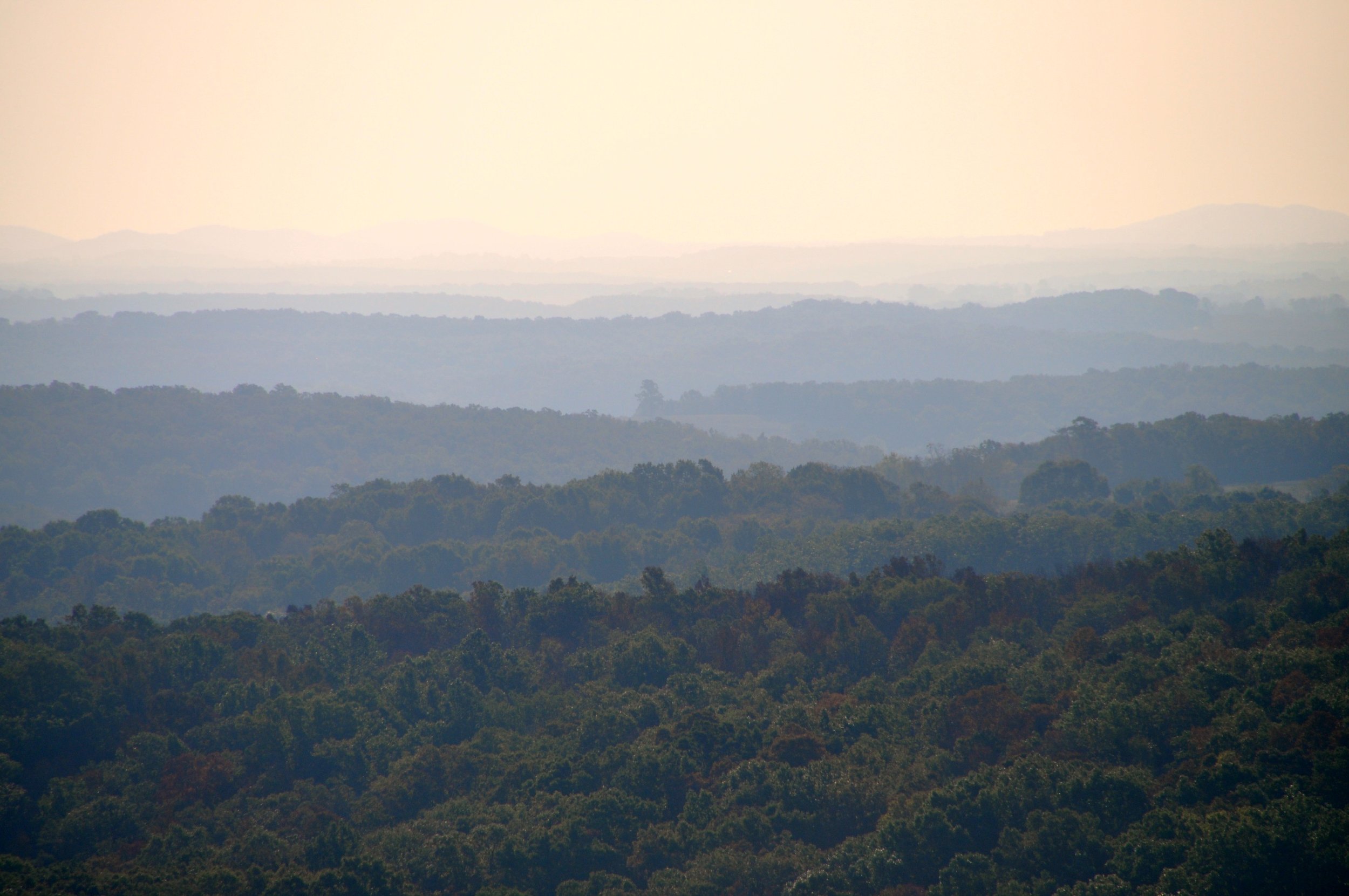The image captures a sweeping long-distance view of what appears to be the Smoky Mountains, showcasing a multi-layered landscape that stretches far into the horizon. In the foreground, a densely forested green mountain stands prominently, covered in vibrant green trees. Behind it, a series of progressively taller and larger mountains fade into the distance, with the furthest peaks barely discernible as light gray outlines due to the misty haze.

The landscape reveals a complex tapestry of undulating hills, valleys, and peaks, presenting at least ten distinct levels of elevation as they recede into the picture. The sky above is a nebulous shade, a blend of gray and white that enhances the fogginess enveloping the distant mountains and casts a faintly ethereal glow over the scene.

As we look closer, the trees are clearly visible with green and brown hues, but as our gaze shifts further out, the details blur, eventually fading into the sky. This sky, described as almost white and very light, adds an airy brightness to the scene, contrasting sharply with the lush greens of the trees and the darker silhouettes of the mountains. The vast expanse of the forest, dotted with a variety of hills, peaks, and valleys, stretches on and on, creating an intricate mosaic of natural beauty. The mist and fog create a sense of depth and scale, emphasizing the grandeur and serenity of this mountainous panorama.